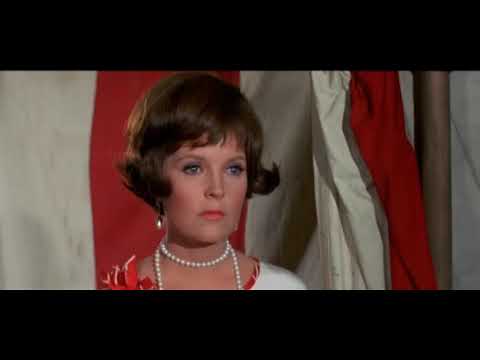The image features a Caucasian woman in her mid-30s, reminiscent of a character from an older TV show or a movie dating back to the 1940s or 1950s. She is shown from the shoulders up, adorned in a sophisticated, period-appropriate style. Her dark to reddish-brown hair is styled in a 1960s fashion, with short, outward-splayed ends that reach her ears and a left-to-right part with bangs. She has blue eyes accentuated with mascara and wears pinkish-red lipstick complemented by blush.

Her attire includes a double-layered pearl necklace; one strand snugly encircles her neck while the second strand drapes down to her chest. Matching dangling pearl earrings complete her elegant look. She is clad in a white blouse featuring a red neckline.

The background reveals a vertically striped white and red flag, possibly part of a tented structure, along with a brown metal pole or flagpole on the right. The image also has large black borders at the top and bottom, suggesting it might be a still from a widescreen movie using early Technicolor technology. The solemn expression on the woman's face, straight nose, and small mouth gives the image a classic, timeless feel.